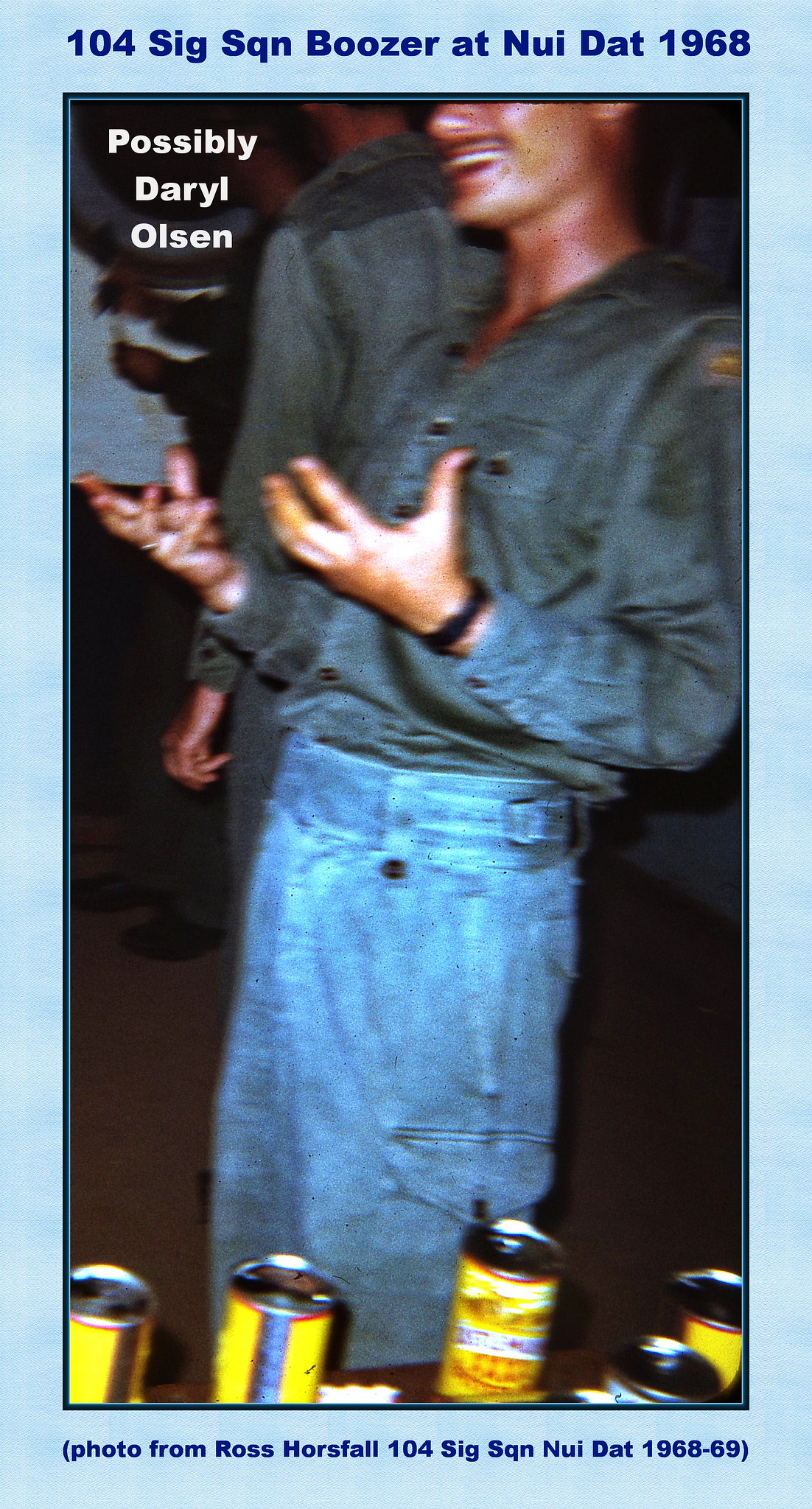The image is a narrow, vertical rectangle, mounted on a light blue background. The photograph itself is darker and features a man visible from his nose down to his knees. He is wearing light blue jeans and a dark shirt or uniform, and has a dark watch on his left wrist. His hands are extended in front of him with the palms up, suggesting a relaxed or casual setting. The man is smiling, and the backdrop includes the partial hand of another individual behind him. At the top of the photograph, there is white text that reads "104 Sig Squadron Boozer at Nui Dat, 1968," indicating a connection to off-duty soldiers in Vietnam. The upper left corner of the image possibly labels the man as "Daryl Olson." Below him, there is a line of yellow, gray, and slightly red cans, likely of beer, some with straws. The image gives off a social, party-like atmosphere, possibly inside a club. The caption also mentions that this photograph is from Ross Horsfall, taken within the period of 1968-69 at Nui Dat, further timestamping and contextualizing the scene.